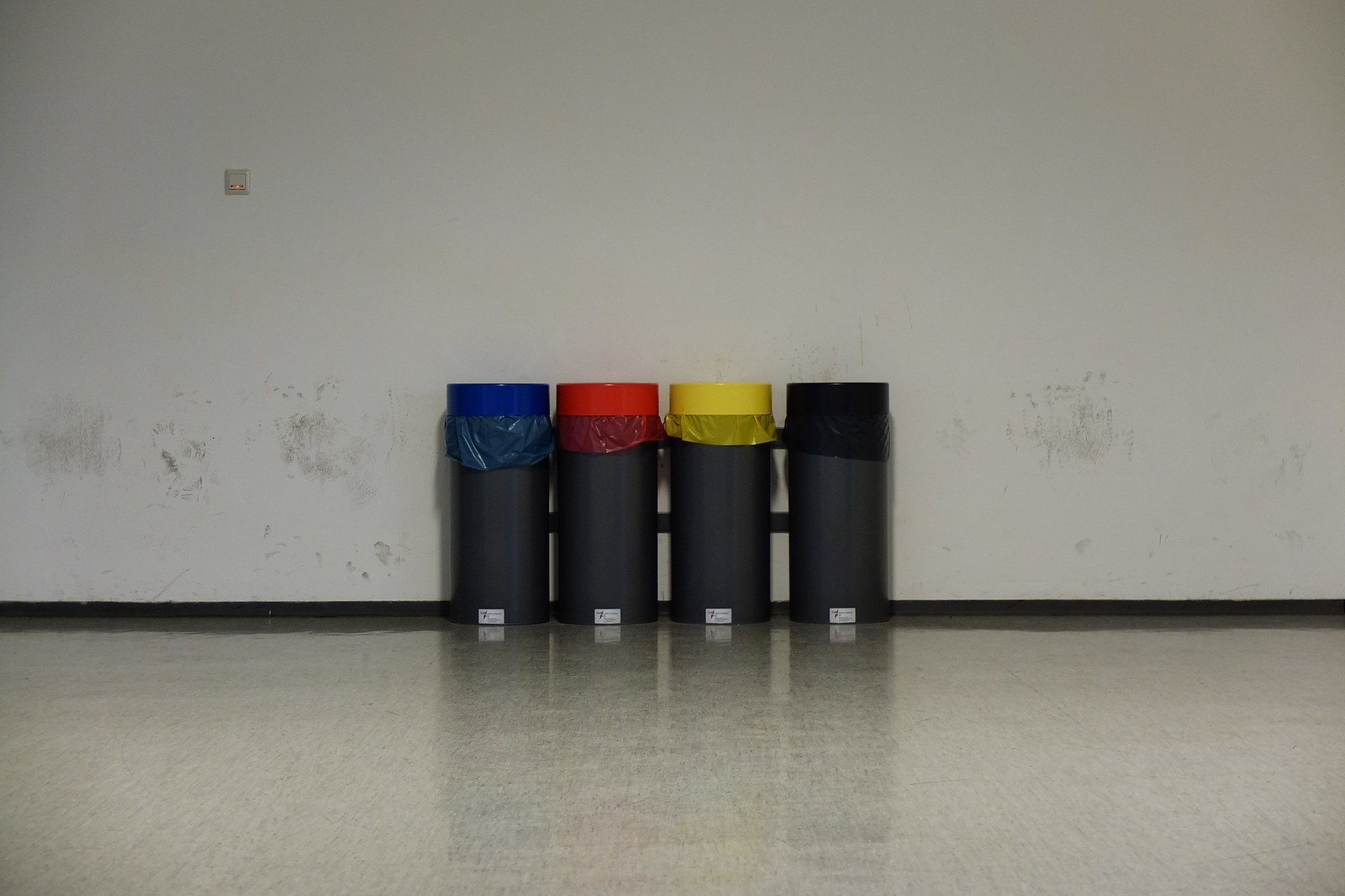This photograph depicts four cylindrical garbage containers lined up against a slightly dirty white wall, which bears scuff marks and other blemishes. Each container is dark gray in color and features a differently colored lid and matching garbage bag that peeks out from the top. Starting from the left, the first container has a blue lid with a blue bag, followed by a red lid with a red bag, then a yellow lid with a yellow bag, and finally, a black lid with a black bag. The containers are placed on a light gray linoleum floor. Additionally, a red light and an unidentified device, possibly a detector, are also attached to the wall above the containers.